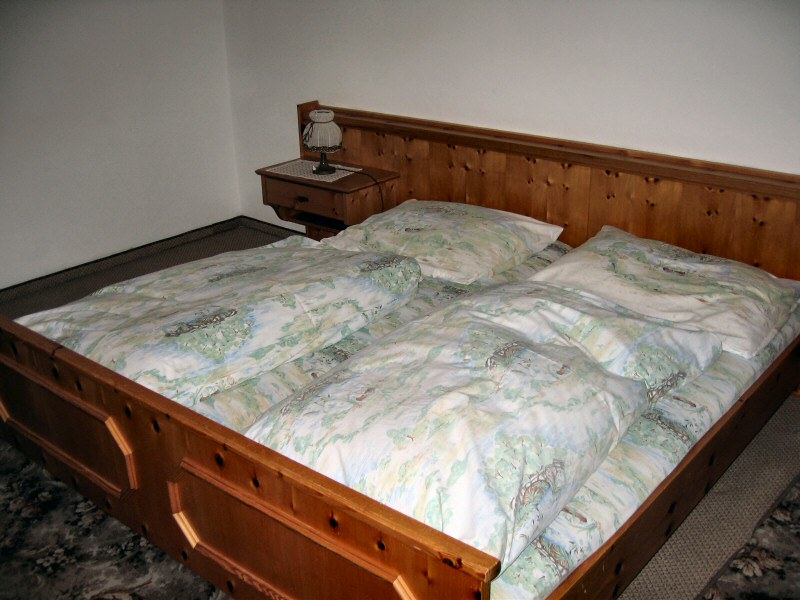This image captures a vintage-themed bedroom, dominated by an older-style double bed made of what appears to be maple wood. The bed features a carved headboard crafted from vertical wood slats, extending beyond the attached nightstands on either side, and a matching footboard with decorative accents. Positioned centrally, the bed accommodates two single mattresses side-by-side, each topped with a neatly folded light blue, green, and white comforter and a matching pillowcase. The room has white walls and is carpeted with a marbleized pattern in gray, white, and cream hues. A small, antique-looking lamp rests on one of the nightstands, which, like the bed itself, is built into the headboard. Heavy shadows envelop parts of the bed, accentuated by the use of flash, giving the room a somewhat dark and amateur photograph feel. There is also a piece of fabric hanging down from behind the side edge of the bed, adding to the snapshot's charm.